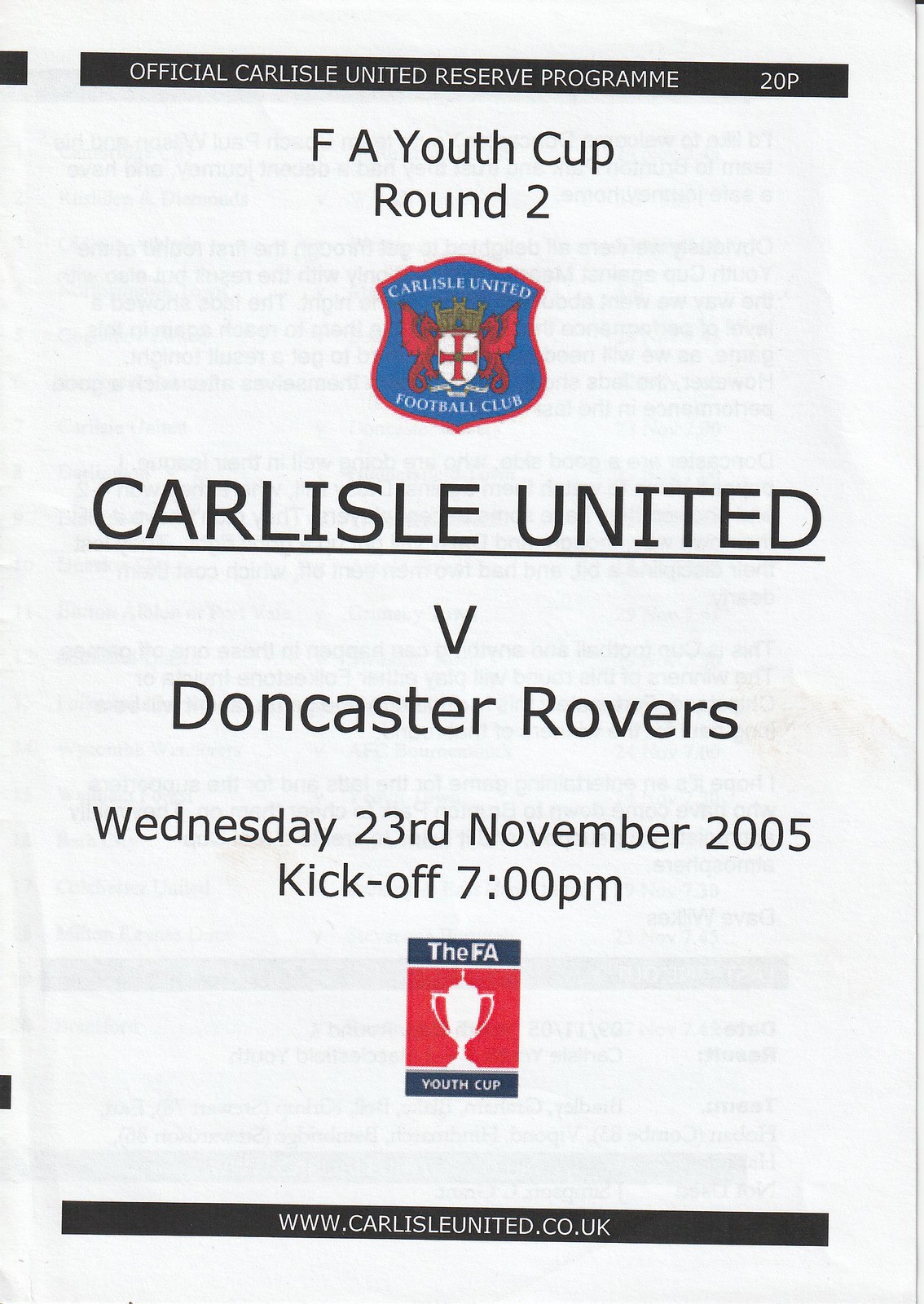This is a color photograph of the official game day program for a Carlisle United Reserve match. The cover features a white background with black text and vibrant logos. At the top, a black bar reads "Official Carlisle United Reserve Program, 20P". Below that, it specifies "FA Youth Cup Round 2". Centrally positioned is the colored insignia of the Carlisle United Football Club, showcasing a shield with griffins and a crown. In large, bold text beneath the logo, it announces "CARLISLE UNITED V Doncaster Rovers" with "CARLISLE UNITED" underlined. Details continue with "Wednesday, 23rd November 2005, kickoff 7 PM". There is also a red and blue FA Youth Cup logo featuring a white trophy icon. At the bottom of the page, a black ribbon holds the club’s website, "www.carlisleunited.co.uk".